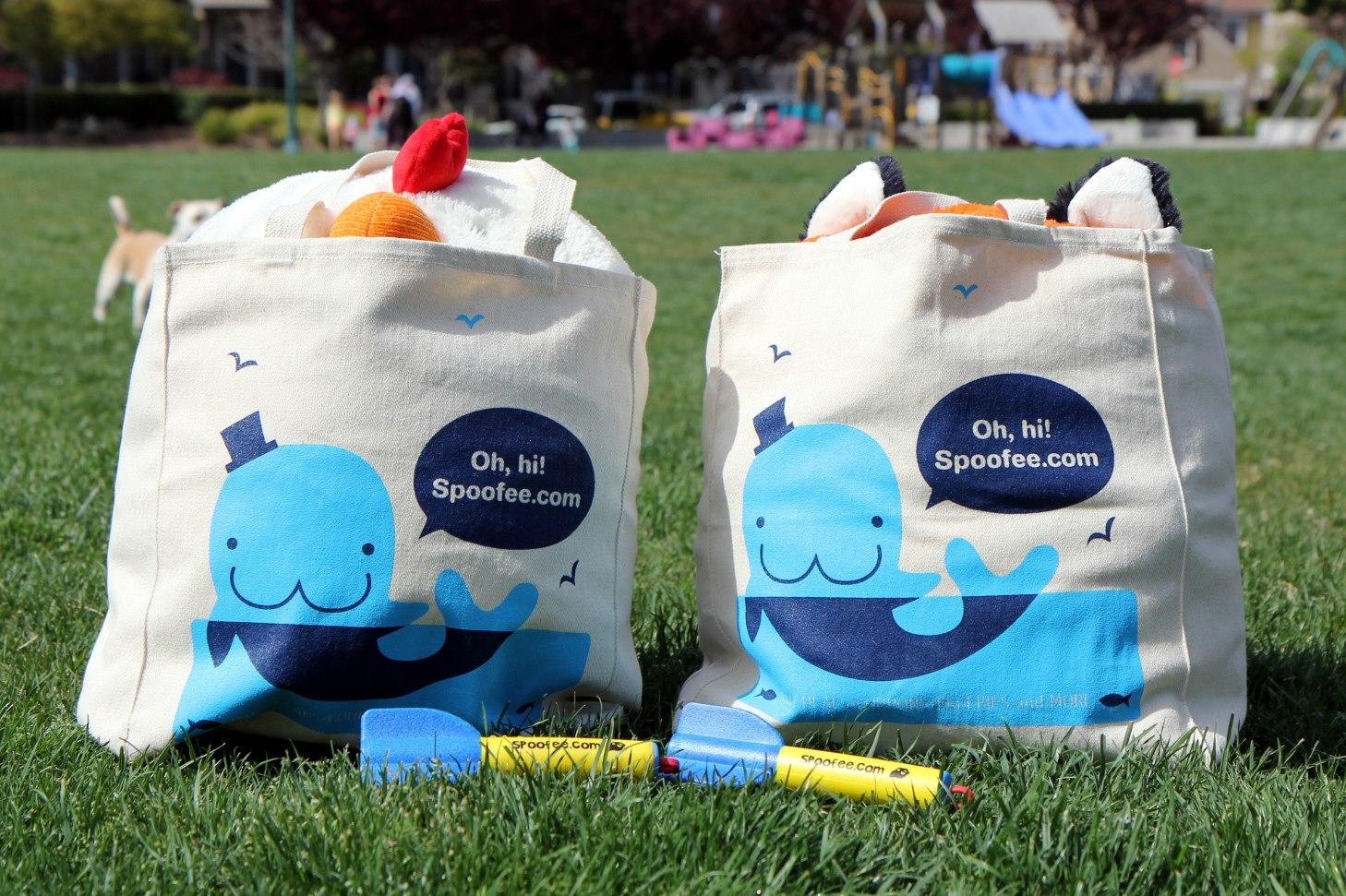In this outdoor image taken at a park, two identical white canvas tote bags are prominently displayed on a grassy lawn. Each bag features a cartoon-style light blue whale wearing a top hat, swimming in matching light blue water, with the lower half of the whale depicted in a darker blue. Above the whale, a dark blue speech bubble reads, "Oh hi, spoofee.com." The bags are filled with stuffed animals, with portions of ears visible at the top—one resembling a chicken with an orange beak and red wattle, and the other possibly a fox or dog with blue and white ears. In front of the bags lie yellow-shafted, blue-finned foam lawn darts, also branded with the spoofee.com logo in blue or black letters. The background reveals a blurred playground featuring blue slides, white rooftops, a pink seating area, people, and a brown and white dog. The scene is set on a sunny day, adding a cheerful ambiance to the image.